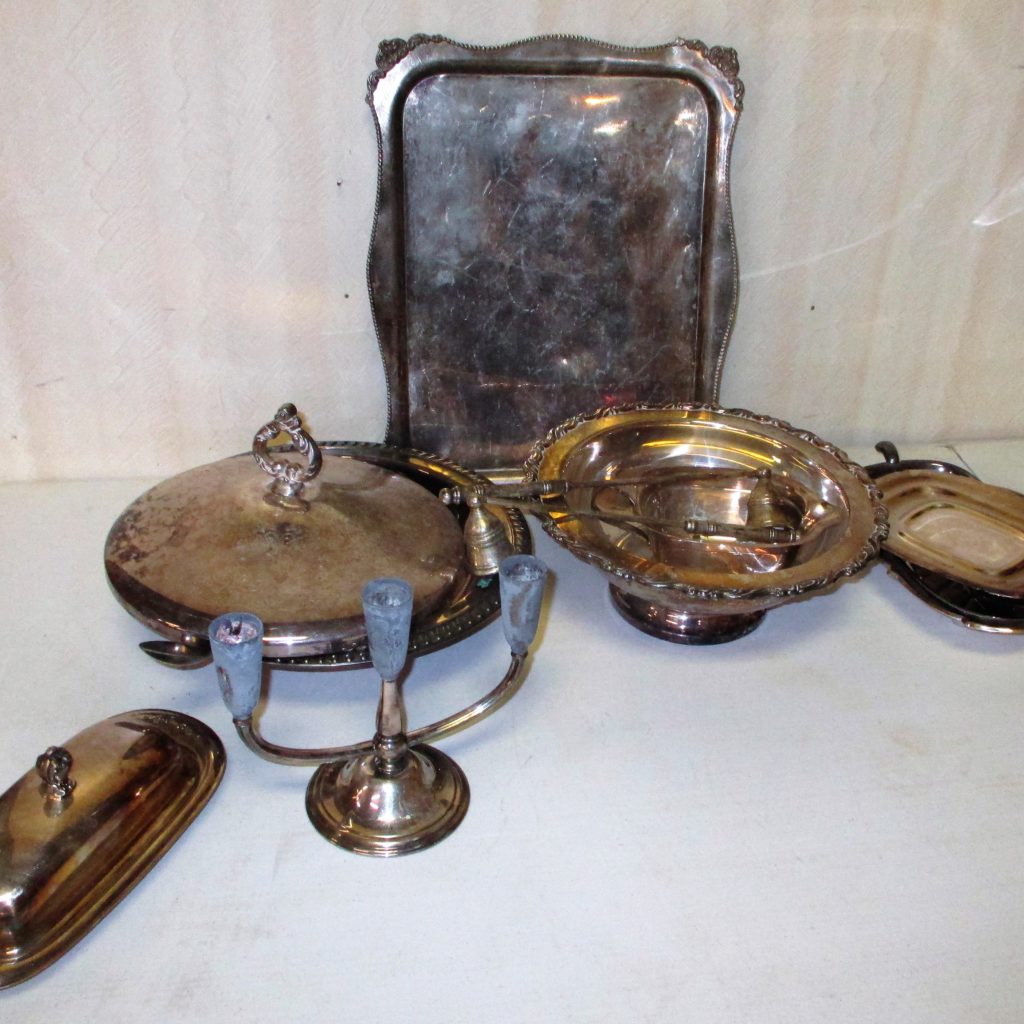The photograph captures an assortment of tarnished silver serviceware arranged on a white surface with a pink and white wall as the backdrop. Dominating the center, we have a large, scratched, and somewhat dirty metal serving tray leaning against the wall. Arranged in front of the tray are various items: a bowl with a pedestal containing a candle snuffer, and a round dish with a lid and handle. Moving to the left side, there's a three-place candelabra designed for tapered candles. Below it is a closed rectangular butter dish, both pieces exhibiting signs of age. On the right side of the image, a couple of open food dishes, one with utensils inside, add to the collection. The color palette features off-white, brown, gold, blue, and deep metallic hues, and the composition of these old kitchen items suggests they are collected on a table or display area.